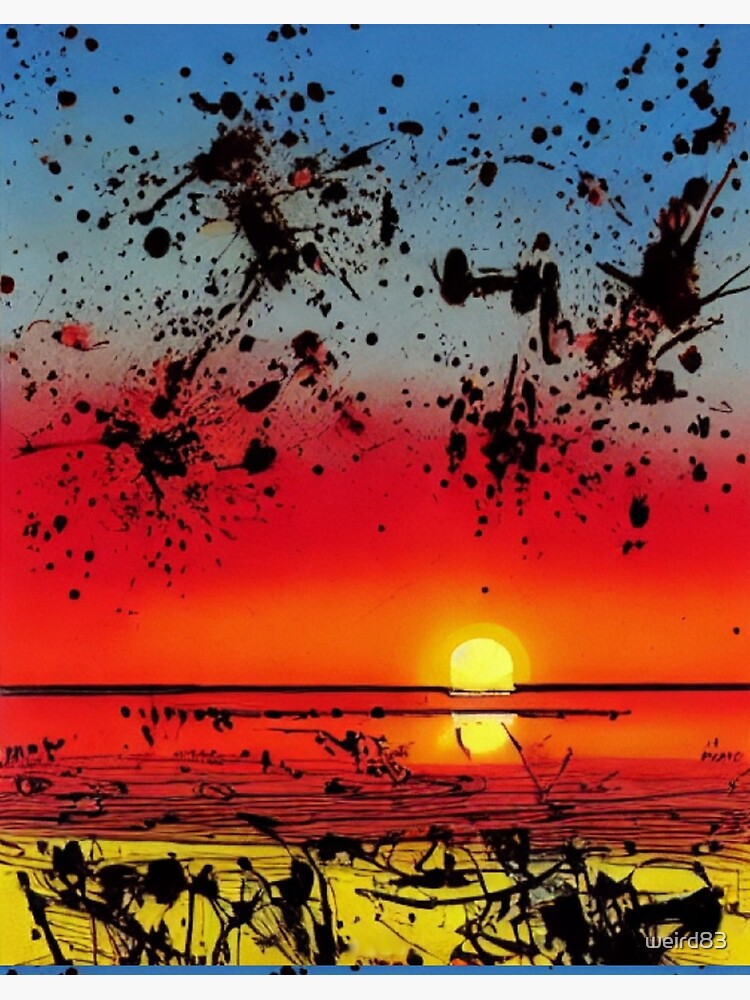The portrait-oriented painting depicts a vibrant and abstract sunset brimming with dynamic color transitions. The lowest part of the background features a strikingly bright yellow strip, which gradually gives way to a vibrant red occupying the middle section of the composition. Above this, the top third showcases a gradient from lighter to a mid-tone blue hue.

Centrally located in the red section is a somewhat uneven horizontal black line, reminiscent of a horizon, with an intensely luminous half-setting sun in vivid yellow sitting atop it. This sun also casts a mirrored reflection below it, forming a yellow circle on the red, almost water-like surface, delineated by another black line. The red area, symbolizing water, displays subtle left-to-right ripples in a slight arc, enhancing its aquatic illusion.

Scattered across the image, primarily at the bottom yellow part and the top blue portion, are random splatters of black paint interspersed with red flecks, seemingly flicked onto the canvas without pattern and adding an additional layer of visual intrigue. Notably, the red section remains free of these splatters, preserving the clarity of the sun and its reflection. This graphic artwork captivates with its bold and eye-catching use of oranges, yellows, and blues, delivering a stylized and digitalized interpretation of a sunset that merges the boundaries of painting and cartoonish render. In the lower right corner, white text reads "WEIRD 83," further accentuating its modern, avant-garde appeal.